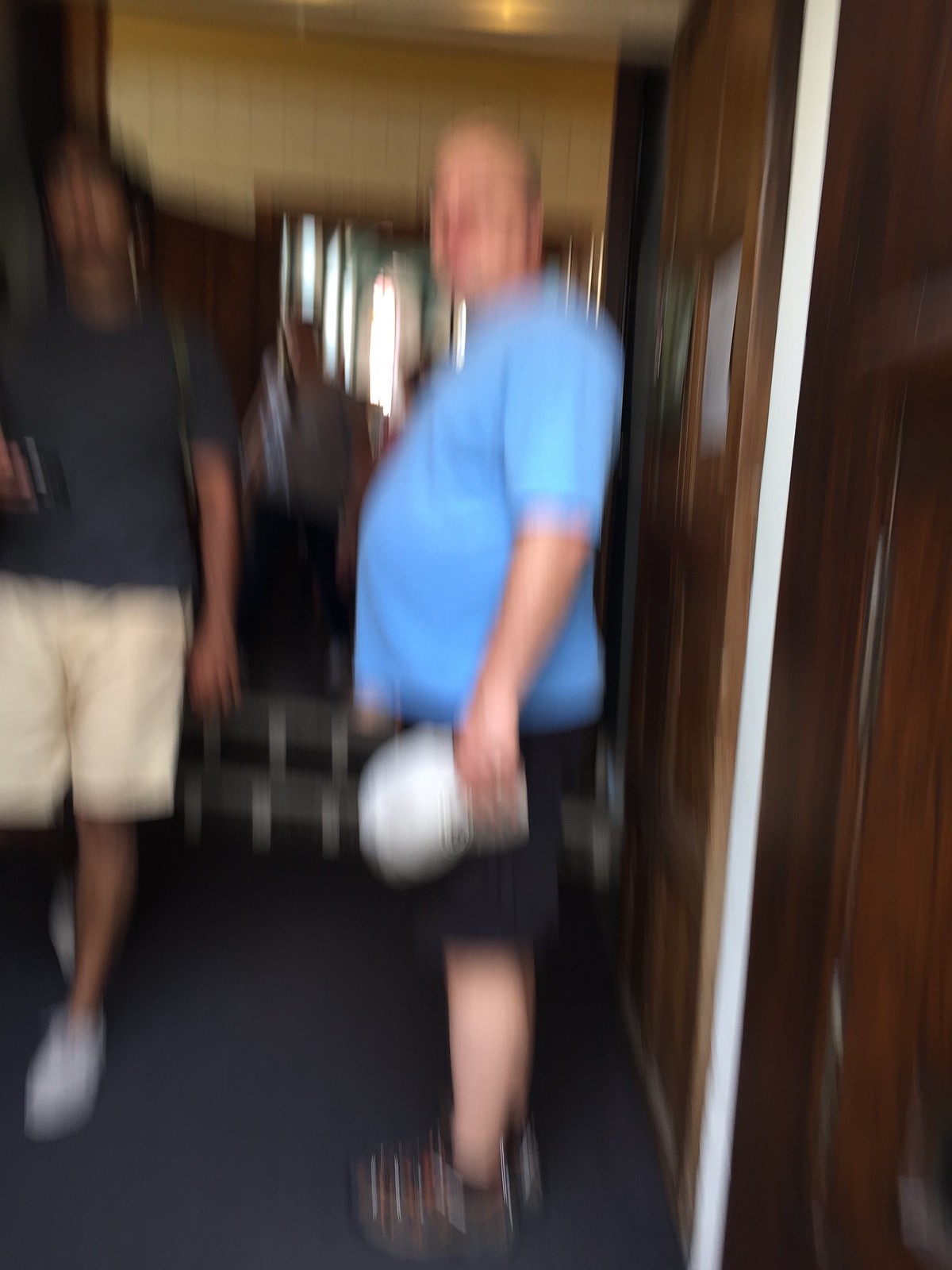In this slightly blurry photograph, the main focus is on two men. Central to the image is a profile view of a man facing left. His face is visible but unfocused. He is wearing a light blue short-sleeve t-shirt that reveals his pot belly, and black shorts. In his left hand, he holds a white baseball cap, and he is shod in dark-colored sneakers. The floor under his feet is a dark gray hue.

To the left side of the image stands another man with dark skin and dark hair. He is dressed in a dark short-sleeve shirt paired with white shorts and white sneakers. 

The backdrop on the right behind the man in the blue t-shirt is a brown wooden wall featuring a white edge, contrasting with the off-white upper background wall and ceiling. Behind both men are two dark steps adorned with white vertical lines on the risers.